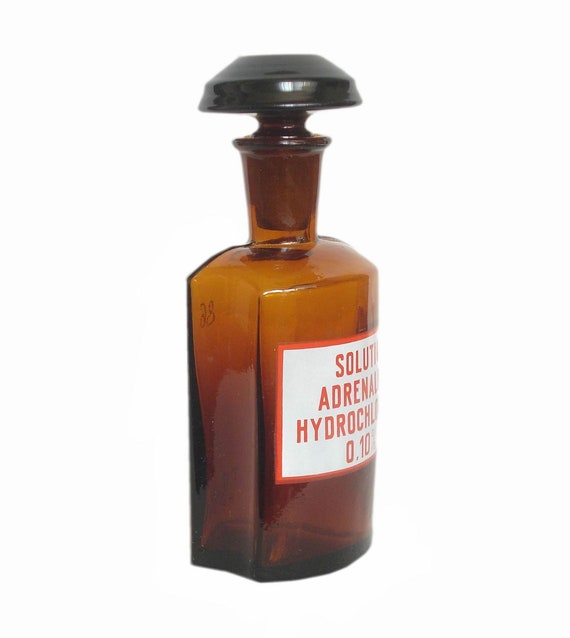This is a highly detailed, portrait-orientation color photograph of a vintage-style amber glass bottle. The setting is minimal, with a stark white background that gives the impression of the bottle floating in space. The bottle itself has an elliptical shape with flat sides and a prominently curved front and back, enhancing its antique aesthetic. It features a tall, narrow neck that flares out at the top, capped with a black, shiny stopper resembling an inverted mushroom or pie shape. A notable detail is the red and white label affixed to the bottle's front, partially obscured, but legible enough to read fragments of the text: "Solution," "Adrenal," and "Hydrochloride," along with the notation "0.10." This label suggests the bottle likely contained a medicinal or chemical solution. The overall style of the image adheres to photographic realism, with a meticulous focus on accurately depicting the bottle's details and texture.